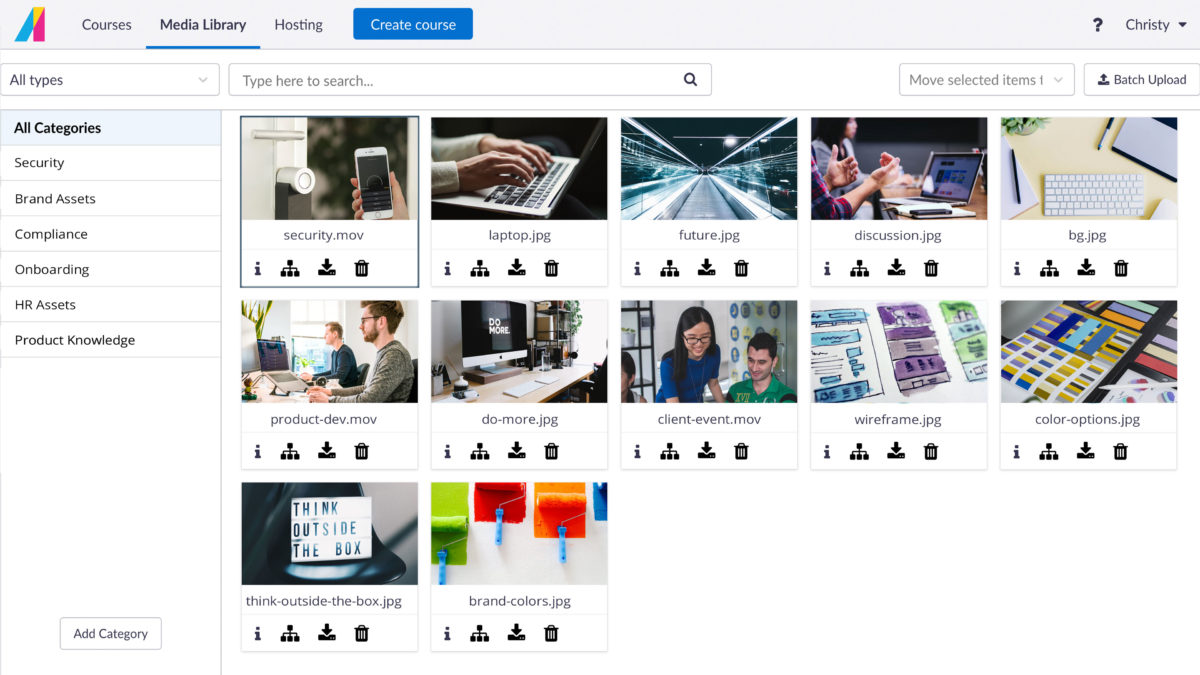On this web page, we see an organized layout starting with a prominent logo to the left. The logo, which resembles the letter "M," is vividly colored in sky blue, yellow, and pink. To the right of the logo are several navigation tabs labeled "Courses," "Media Library," and "Hosting." Adjacent to these tabs, there is a distinctive blue button that reads "Create Course." Additionally, there's a question mark icon and a drop-down arrow beside the user name "Christy."

On the left side of the page, beneath a section labeled "All Types" with its drop-down arrow, the "All Categories" option is highlighted. This section includes a list of categories such as "Security," "Brand Assets," "Compliance," "Onboarding," "HR Assets," and "Product Knowledge." At the bottom of this list, there's an "Add Category" button available.

Moving to the main section of the page, there's a search box labeled "Type Here to Search," and to its right, a "Move Selected Items" function with a drop-down arrow, followed by a "Batch Upload" button.

The primary content consists of 12 photographs. Here are their details:
1. The first photo features a person holding a smartphone.
2. The second image shows someone typing on a laptop keyboard.
3. The third image is labeled "Future" and appears to be tech-related.
4. The fourth image, named "Discussion," depicts a group of people in a conference room and is a JPEG file.
5. To its right, there's a picture of a computer keyboard alongside writing tablets and pens.
6. Below, an MOV file named "Product" shows two men at a table with computer screens, seemingly in an office setting.
7. Next, a JPEG shows a computer monitor on a desk.
8. An MOV file captures a woman instructing a man, possibly in an office environment.
9. The following JPEG is unclear in subject.
10. Another JPEG appears to depict a colorful book.
11. Near the bottom, a JPEG highlights the phrase "Think outside the box."
12. The final image is a JPEG showing colorful envelopes mounted on a wall.

Each of these images includes icons for information, download, trash, and one unidentified icon, indicating possible actions that the user can take for each image. This detailed layout and the variety of content available provide a comprehensive overview of the web page.